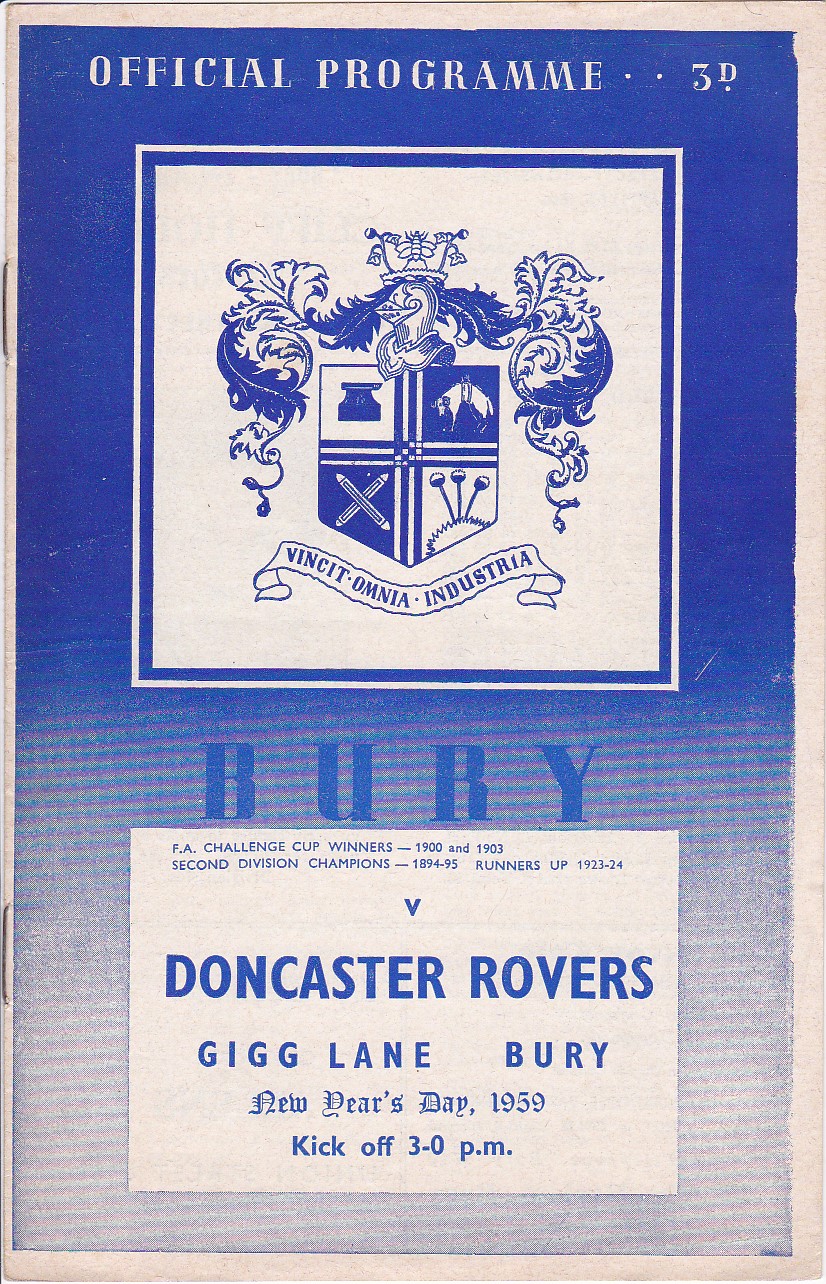This image depicts the cover of an official program for a Doncaster Rovers football match held on New Year's Day 1959 at Gig Lane, Bury, with a kickoff time of 3 p.m. The top of the program is adorned with bold white lettering that reads "Official Program" in 3D formatting, against a deep blue background that gradually fades into a lighter color towards the bottom. Central to the design is a prominent square featuring the Doncaster Rovers coat of arms, which includes intricate medieval imagery: a helmet surrounded by feathers, a suit of armor, an anvil, two crossed swords, and other less discernible elements. Beneath the coat of arms is a banner inscribed with the Latin motto "Vincit Omnia Industria" (Industry Conquers All). Below this, additional text details the occasion as a Challenge Cup match. Further down, a white rectangle contains smaller lettering providing more specifics about the event.